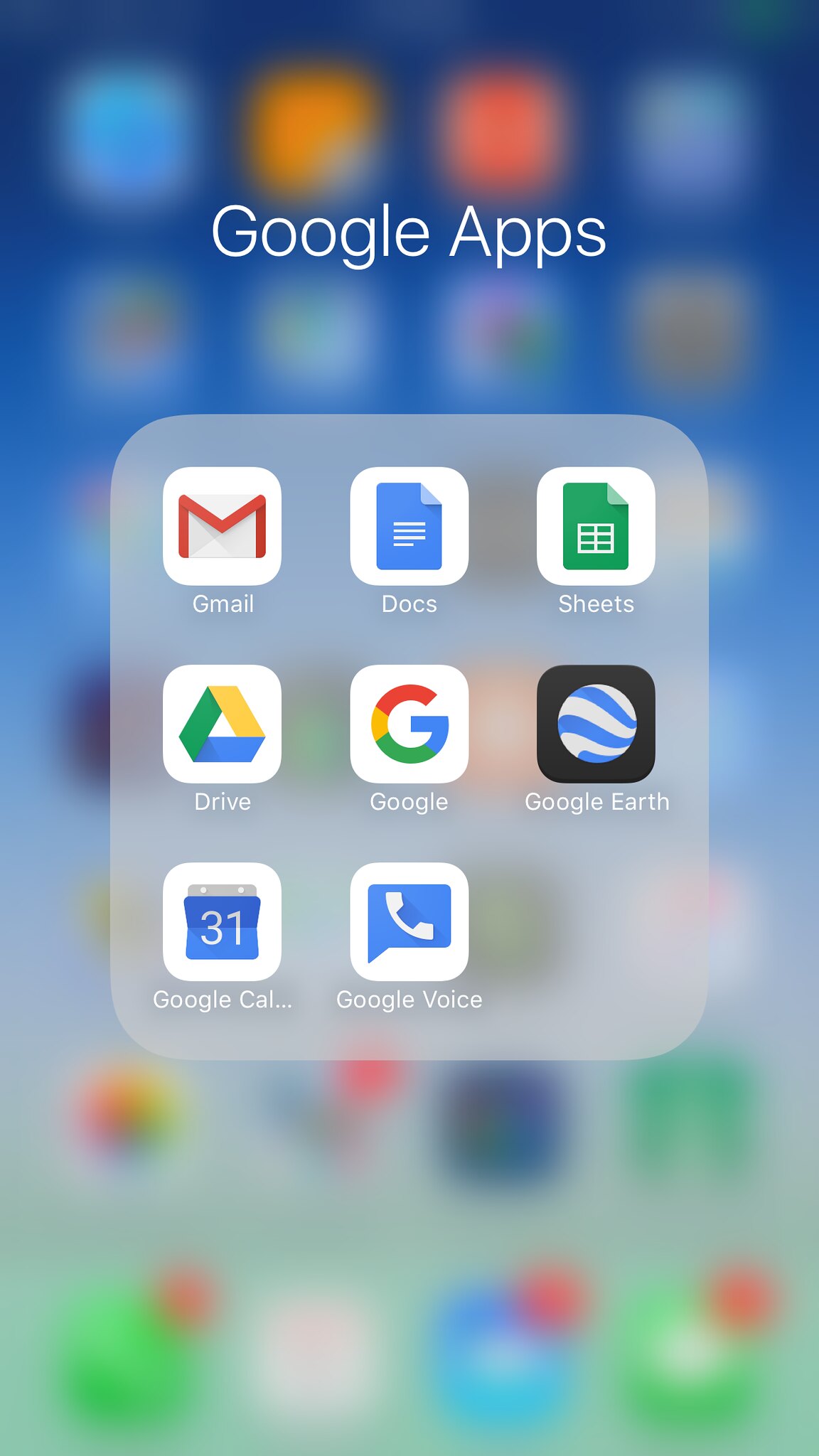This image showcases the screen of a smartphone featuring a distinctive user interface. The background displays a gradient that transitions from a deep blue at the top to a paler blue and ultimately a hint of green at the bottom. Overlaying this background is a grid pattern composed of rounded square dots arranged horizontally in rows of four.

Prominently placed at the top of the screen are the words "Google Apps" in bold, white text. Dominating the center of the screen is a large, square panel with rounded edges. This panel is semi-transparent, revealing a subtle outline of the background behind it. 

Within this translucent gray panel, app icons are neatly organized. The top two rows each contain three icons, while the bottom row consists of two icons. The apps displayed include:

- Gmail
- Docs
- Sheets
- Drive
- Google
- Google Earth
- Google Calendar
- Google Voice

Each icon is visually consistent, maintaining a cohesive design typical of Google's branding.